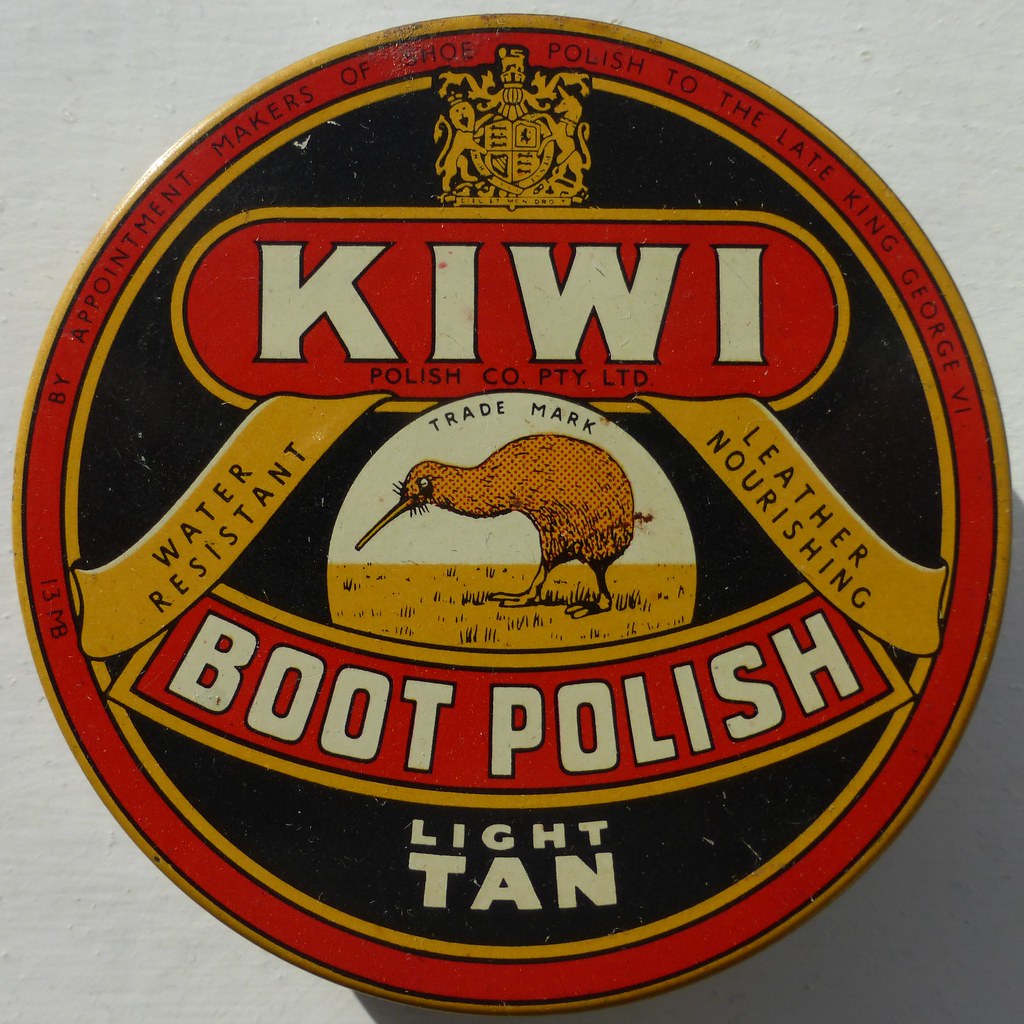This image depicts the top view of a Kiwi boot polish can, showcasing its intricate and colorful design. The can is circular, bordered by alternating gold and red outlines, with a predominantly black background that accentuates the vibrant elements. 

At the top, the word "Kiwi" is prominently displayed in bold white letters against a red backdrop bordered in gold. Beneath this, in smaller black lettering, it reads "Polish Co Pty Ltd." Above the Kiwi logo, there is a gold symbol featuring two animals flanking a shield, reinforcing the brand's regal heritage. Extending from the symbol are two gold banners; the left one reads "water resistant," and the right one reads "leather nourishing," both in black letters.

Central to the design, under the Kiwi logo, is a gold-colored bird, presented as the trademark, with its beak pointed towards the left. The word "Trademark" arches above this avian symbol. Below the bird, in a red banner, it says "boot polish" in white letters. Further down, in a black section at the bottom of the can, it states the polish color: "light tan" in white letters.

Encircling the can, a red border features the statement: "By appointment, makers of shoe polish to the late King George VI," a testament to the brand's legacy and quality. The overall design elements are predominantly in white, red, gold, and black, creating a visually striking and detailed appearance designed to denote sophistication and trust in the product's effectiveness and heritage.